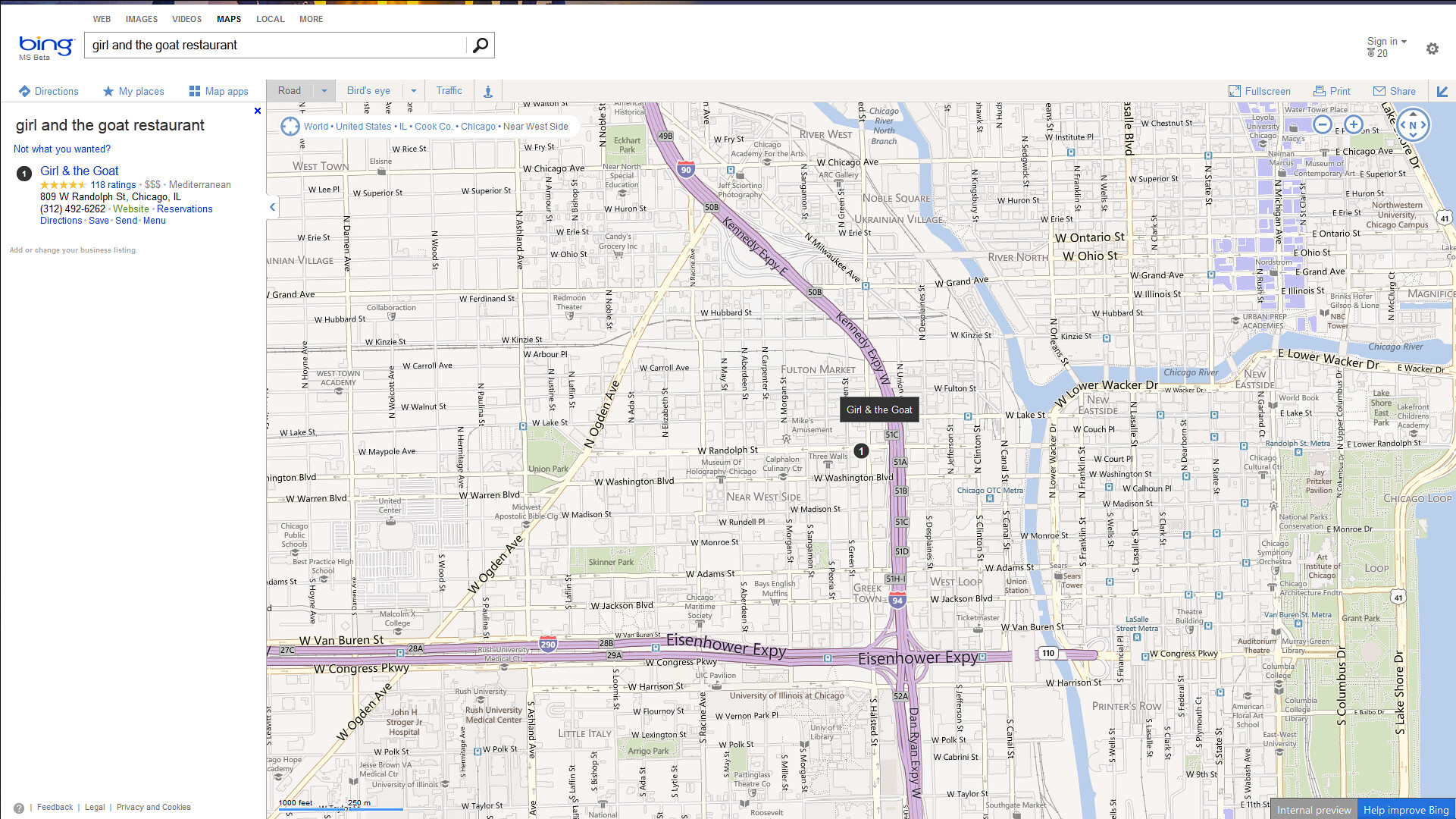This color photograph appears to be a screenshot taken from a web page. In the top left corner, there is a clean, blue-styled logo of a search engine named "Beam." Beside it is a search bar where "Girl and the Goat Restaurant" has been entered, followed by a magnifying glass icon indicating the search function. The search has been executed, resulting in a street map displayed below.

The map features a black highlight on the location of the "Girl and the Goat" restaurant, situated conveniently near an interstate highway. Although the map itself is not highly detailed—making much of the smaller text illegible—it includes several larger, more readable place names that identify different locations within the city.

On the left side of the image, the search result includes a clickable hyperlink labeled "Girl and the Goat Restaurant," along with an address. Despite the text being somewhat blurry, "Chicago, Illinois" is discernible, confirming the location within the city. Overall, the map provides a visual context for the restaurant's exact position in Chicago, offering users a snapshot of its geographical setting.